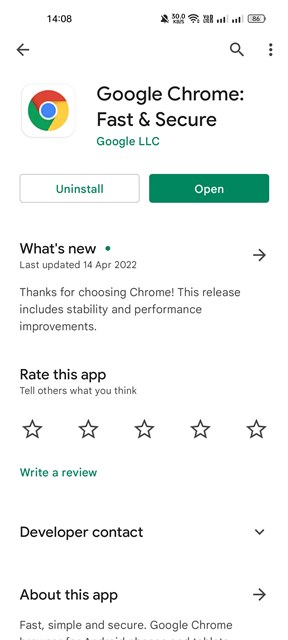The image is a screenshot taken from a cell phone. The background is entirely white. In the top left corner, the time is displayed as 14:08. In the top right corner, there are several icons: a notification bell with a line through it, an unreadable symbol associated with the number 30.0, a full Wi-Fi signal icon, an unidentified icon, two cell phone signal strength indicators both displaying four out of five bars, and a battery icon showing 86% remaining charge.

Below these icons, there is a navigation bar with a back arrow on the left and a search icon followed by three vertical dots on the right. Underneath this bar, the Google icon is displayed alongside the text "Google Chrome: Fast & Secure," with "Google LLC" written beneath it. 

Following this, there are two buttons: one with a white background and green text labeled "Uninstall," and another with a green background and white text labeled "Open." 

Further down, the section titled "What's New" indicates that the app was last updated on April 14th, 2022, with a right arrow icon beside it. Below this, a message reads "Thanks for choosing Chrome. This release includes stability and performance improvements."

Additionally, there are sections for rating the app, developer contact information, and details about the app itself at the bottom of the screenshot.